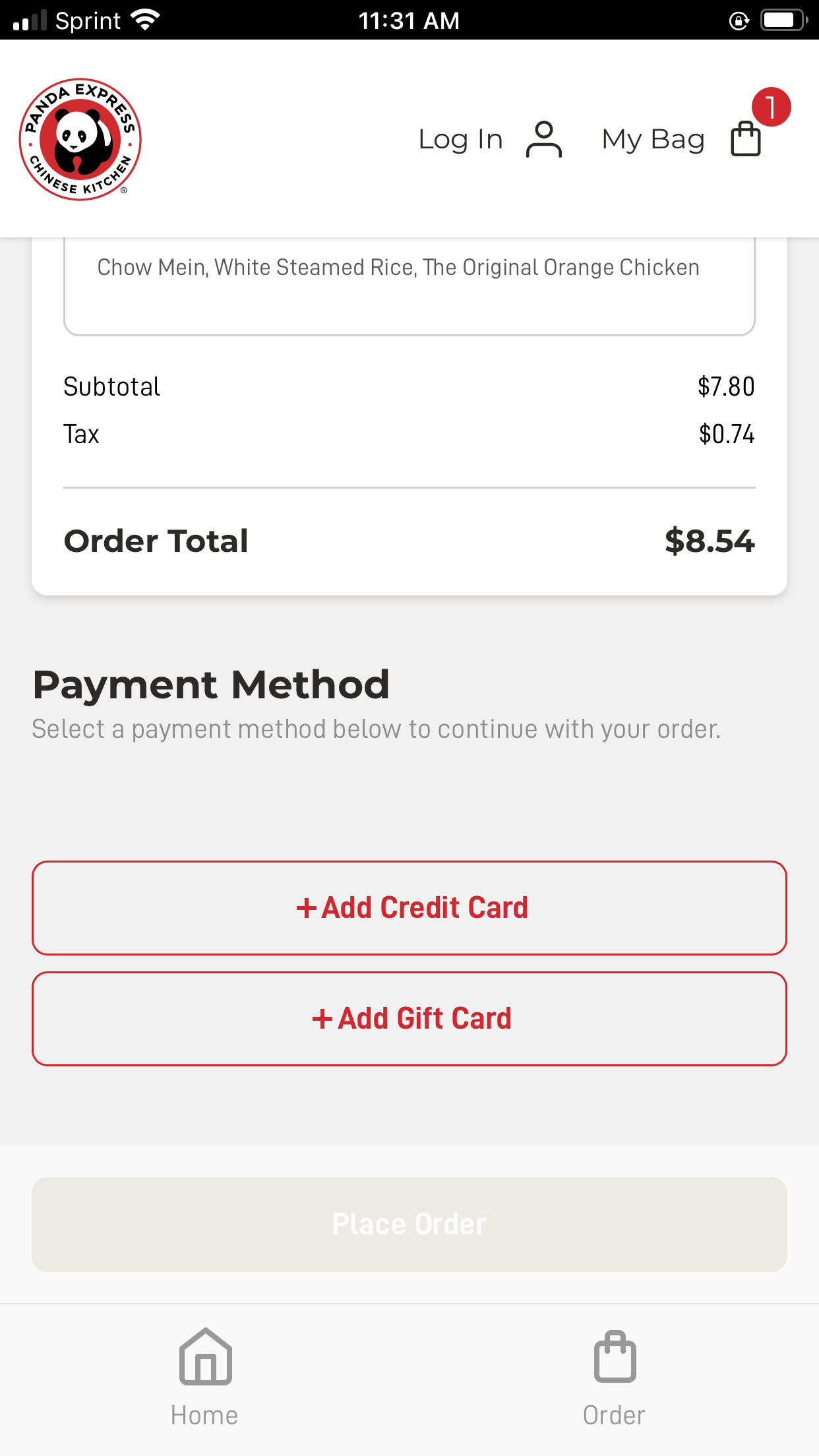This image is a screenshot displaying a mobile device screen, with a black status bar running along the top portion. The status bar shows partially connected network signals with only two bars active, accompanied by a full Wi-Fi indicator. The current time is indicated as 11:31 a.m., alongside a battery icon. Further below, a Panda Express logo featuring a panda is visible.

The main content of the screenshot captures a mobile ordering interface for Panda Express. The screen text includes a message prompting "Look in my bag," followed by the listed items: "Chow Mein," "White Steamed Rice," and "The Original Orange Chicken." The pricing details are also visible, with a subtotal of $7.80, tax amounting to $0.74, and an order total of $8.54.

Following the pricing segment, there is an instruction to "Select the payment method below to continue with your order," with options to "Add to Cart" and "Add Gift Card." The "Place Order" button is noticeably blurred. The options "Home" and "Order" are also present, likely as navigation buttons.